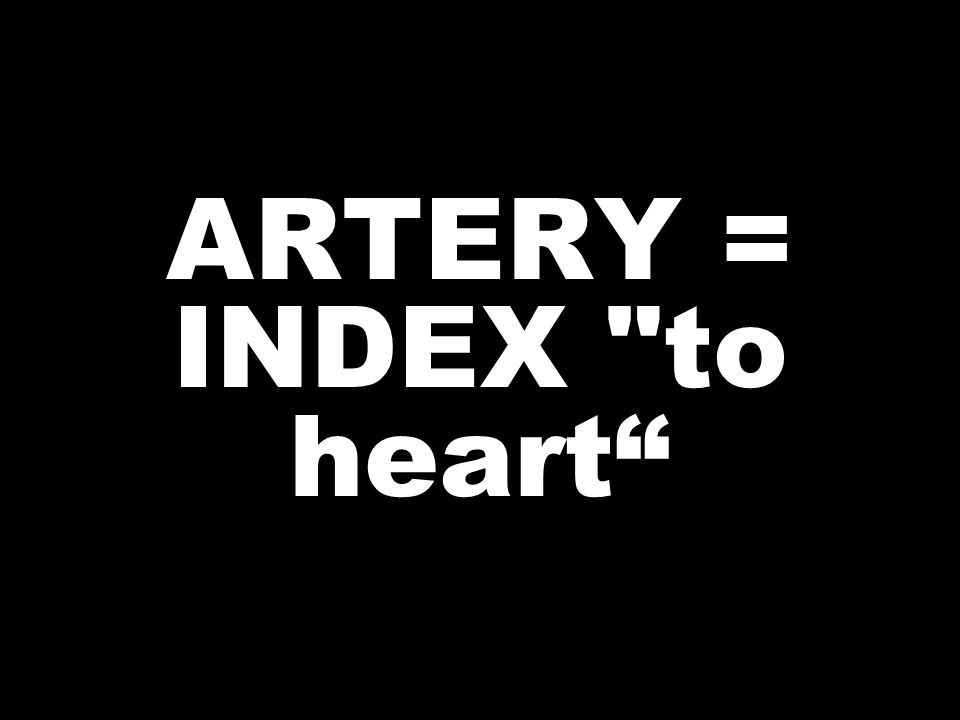The image features a square black background with stark white, centered sans-serif text in three lines. The first line presents the word "ARTERY" in uppercase, followed by an equal sign. The second line reads "INDEX," also in uppercase, followed by a lowercase "to" enclosed in white quotation marks. The third and final line displays the word "heart" in lowercase, ending with a quotation mark. The overall message conveyed is "ARTERY = INDEX 'to heart'."